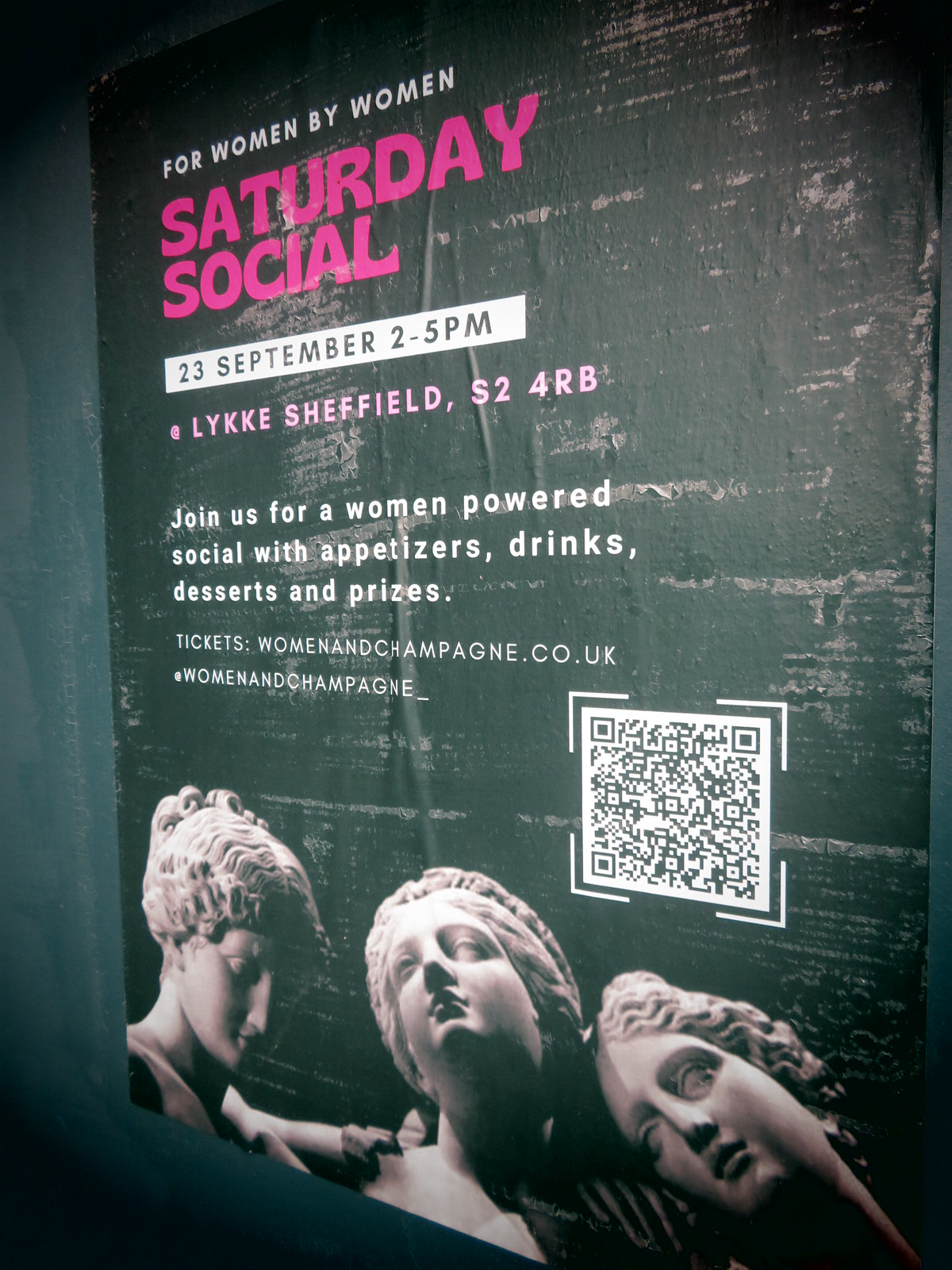The poster is a black advertisement banner for an event called "Social Saturday by Women for Women, 23rd September from 2 to 5 p.m. at Lake Sheffield." It prominently features three busts of women that resemble Greek statues positioned at the bottom of the banner. The statues’ heads, with hair styled in intricate updos with many curls, show various expressions: one has eyes closed with her head tilted down, the middle one looks up towards the sky, and the third rests on the middle one's shoulder, gazing outward. None of the statues are smiling.

The text on the poster is in pink and white, encouraging attendees to join for a woman-powered social event with appetizers, drinks, desserts, and prizes. At the bottom, there's a QR code for tickets, with the website listed as womeninchampagne.co.uk. The design places the statues below the text, creating a captivating visual contrast against the black background.